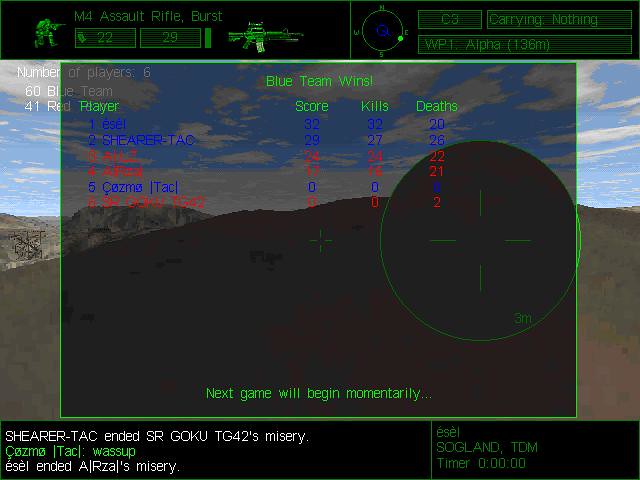This detailed screenshot from a video game showcases the end screen of a match, providing an in-depth look at various game elements and player statistics. At the top, a black rectangle features a crouching soldier, equipped with a backpack and an M4 assault rifle set for burst fire. The soldier's silhouette and accompanying text, including "M4 Assault Rifle Burst," are highlighted in lime green. Adjacent to this, two small green rectangles display ammunition counts, marked as "22" and "29," alongside an M4 rifle silhouette and a lime green bar.

To the right, there's a map indicating cardinal directions with a "Q" in the center. Additional green rectangles provide more details: one displays "C3," and another states "carrying nothing." Below these, it reads "WP1 Alpha (136M)," specifying a waypoint 136 meters away. The game's player count is noted with "6 60 blue team 41 red team white."

At the bottom of the screen, a black rectangle features player interactions in lime green text, such as "SHEARER-TAC ended SRGokuTG42's misery" and "ESEL ended Alraza's misery." Accompanying this is the leaderboard, showing detailed player statistics, including names, scores, kills, and deaths:
- ESEL (Blue) - Score: 32, Kills: 32, Deaths: 20
- SHEARER-TAC - Score: 29, Kills: 27, Deaths: 26
- ALZ - Score: 24, Kills: 24, Deaths: 22
- AFAZL (Red) - Score: 17, Kills: 16, Deaths: 21
- COSMOTAC000 and SRQJQU002 are also listed with their respective statistics.

The background scenery appears to depict a hilly or desert landscape under a blue sky, typical of a first-person shooter environment. The overlay hints at the imminent start of the next game, creating an immersive and competitive atmosphere.